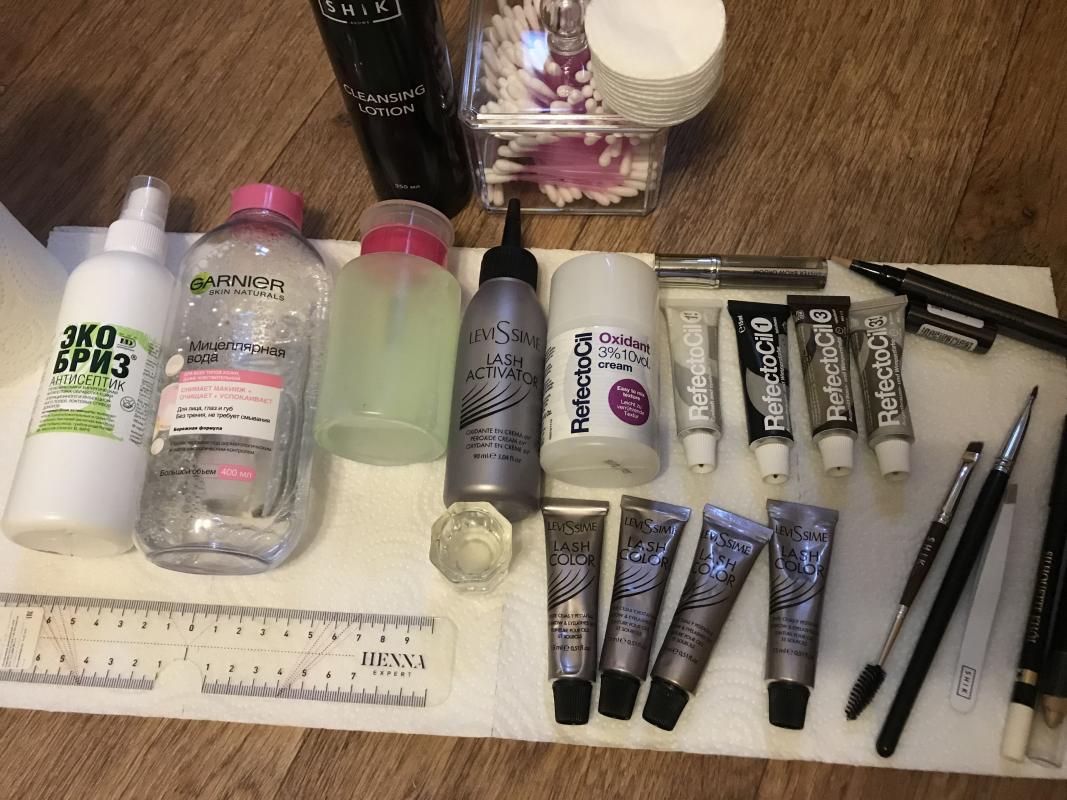A meticulously organized display of various cosmetics and beauty products arranged on a wooden table. At the top of the image, Q-tips and cotton swabs are neatly placed, with the cotton swabs stored in a small container. To the left, there is a bottle of cleansing lotion. Below these items, an array of products is systematically laid out on paper towels.

From left to right, the arrangement begins with a spray bottle followed by a Garnier facial cleanser or micellar water. Next is a pump bottle, possibly containing polish remover, and beside it is a squirt bottle labeled as a lash activator. Continuing along, there's a facial cream branded as Refactosil, and four tubes that appear to be foundation.

To the right side, a selection of brushes and utensils are carefully placed, including tweezers and various tools for applying eye shadow and lashes. At the bottom, there's a collection of lash colors, indicating that this assortment is prepared for detailed eyelash attachment and enhancement activities.